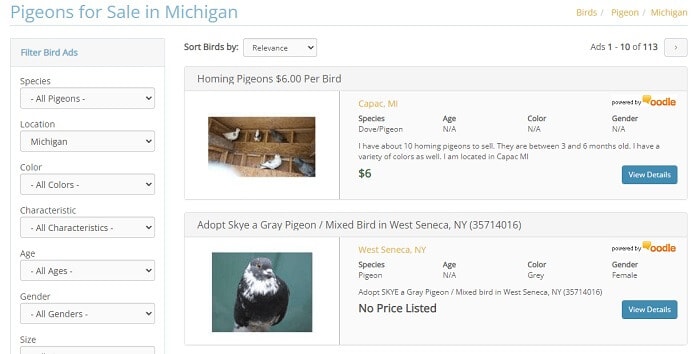This is a webpage dedicated to pigeons for sale in Michigan. At the top of the webpage, displayed in light blue text, is the heading "Pigeons for Sale in Michigan." On the far right of the page, in smaller gray text, it reads "Birds / Pigeons / Michigan." 

To the left side of the screen, there are filtering options presented in a vertical rectangular box with a gray background. The box is titled "Filter Bird Ads" and includes various categories for filtering: Species, Location, Color, Characteristic, Age, Gender, and Size.

On the right, there are two main selections. The first is highlighted by a gray banner across the top that states, "Homing Pigeons, $6 per bird." Below this banner, written in light gray text, is a brief description: "I have about 10 homing pigeons to sell. They are between three and six months old. I have a variety of colors as well."

The second option features another gray banner that reads, "Adopt Sky, a gray pigeon, mixed bird in West Seneca, New York." Accompanying this text is a picture of the pigeon named Sky. Below the image, inside the same box, is the detailed description: "Adopt Sky, a gray pigeon/mixed bird in West Seneca, no price listed."